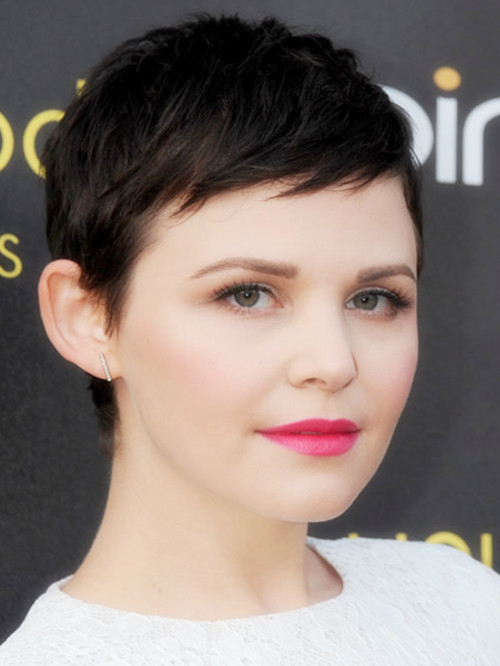The photograph is a close-up of a stunning young woman, potentially in her late 20s to early 30s. She has an exceptionally short, boyish cut of brown hair, meticulously styled to the side. Her striking green eyes are accentuated with mascara and possible false eyelashes, and her makeup gives her a flawlessly smooth complexion. Her lips are adorned with a vivid pink lipstick. She is wearing tube-shaped earrings in her right ear and a white blouse embellished with an embroidered floral pattern, though the photo is cropped from her chest down. The backdrop is a black wall featuring a smattering of yellow and white text, partially obscured by her head, with discernible letters "I-N" on the right side. The photograph primarily captures her face, highlighting her natural beauty and poised elegance.